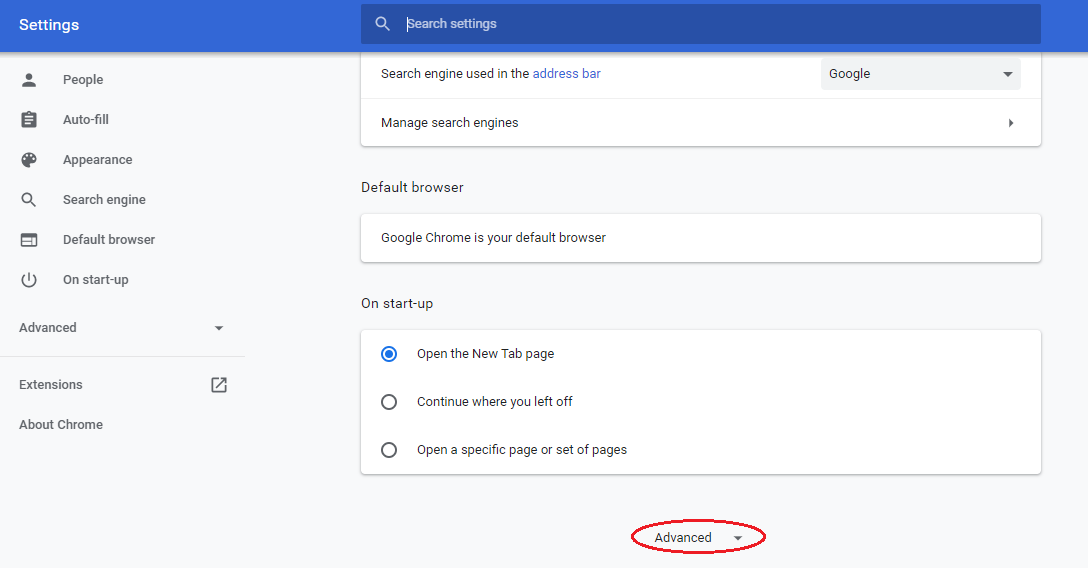The image depicts a computer settings screen in a landscape format. At the top, a blue bar stretches across the width of the screen, and in the top left corner, the word "Settings" is displayed in white. Approximately one-third of the way across the top bar, there is a dark blue search bar containing a white magnifying glass symbol and the text "Search settings."

Below the top bar, a column on the left side of the screen lists various settings categories, each accompanied by an icon. From top to bottom, the categories and their respective icons are as follows:
1. A person icon labeled "People."
2. A clipboard icon labeled "Auto-fill."
3. A paint palette symbol labeled "Appearance."
4. A magnifying glass icon labeled "Search engine."
5. A browser icon labeled "Default browser."
6. A power button icon labeled "On startup."

Below these categories, still in the left column, there is an "Advanced" option indicated by a drop-down arrow, followed by "Extensions" and "About Chrome."

To the right of the left column, under the search bar labeled "Search settings," there are two columns displaying further details. The top section in a white bar contains options for the "Search engine used in the address bar," with "Google" as the selected option, featuring a drop-down menu next to it. Below this, there is a "Manage search engines" option, which has a right-arrow icon.

The background then transitions to grey, where the "Default browser" section indicates that "Google Chrome is your default browser" inside a white block. Continuing downward, in the "On startup" section, the first circle checkbox is filled with a blue dot, indicating the selection of "Open the New Tab page." The other options available but not selected are "Continue where you left off" and "Open a specific page or set of pages."

At the very bottom, centered in the two columns under the "On startup" section, there is another "Advanced" option, including a drop-down arrow, circled in red.